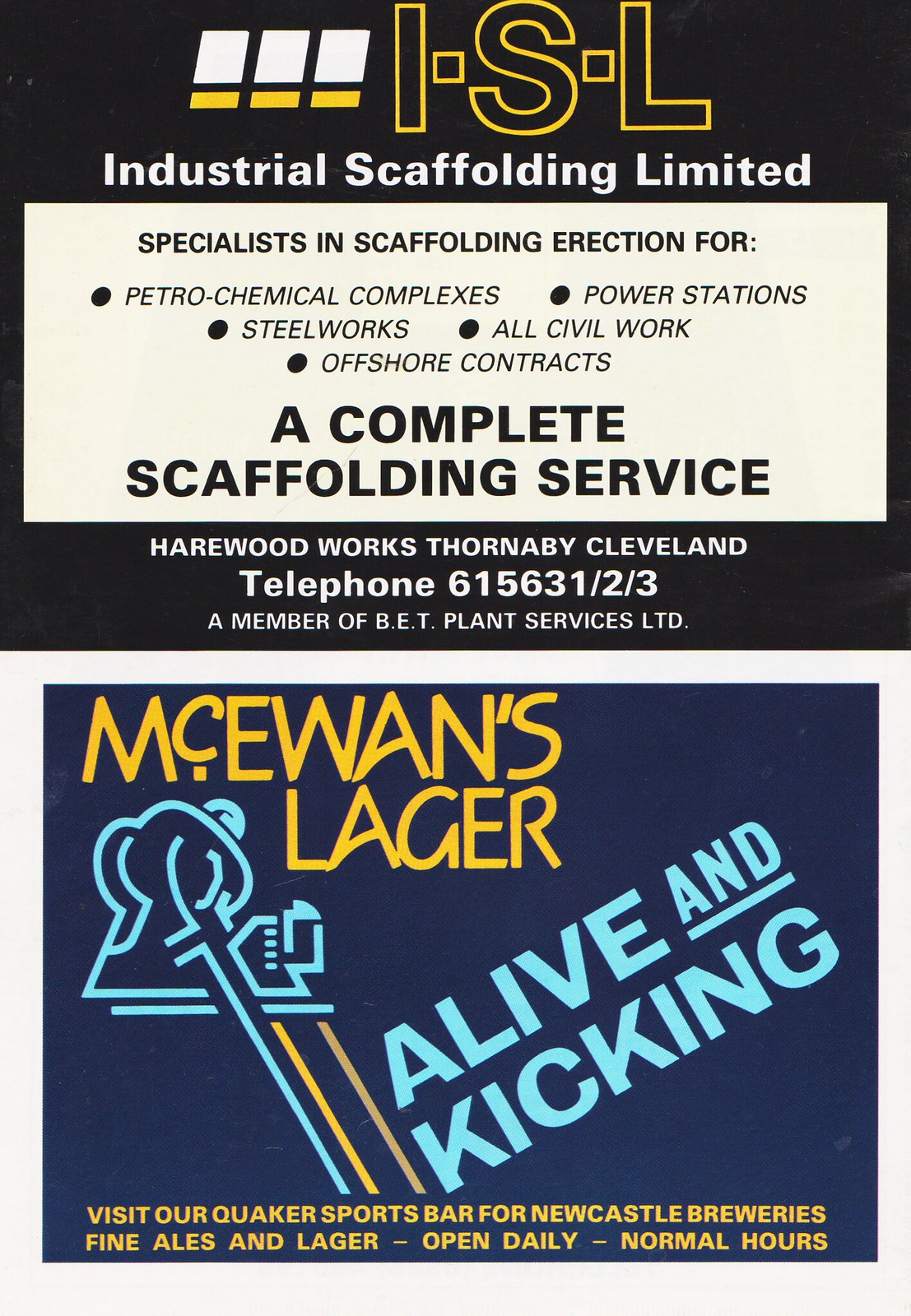The image features two stacked advertisements, showcasing distinct businesses. 

The top advertisement, set against a black background, highlights "ISL Industrial Scaffolding Limited," with "ISL" prominently displayed in yellow. The ad details the company's expertise in scaffolding erection for various sectors, including petrochemical complexes, power stations, steelworks, civil works, and offshore contracts, all categorized with bullet points. It emphasizes that they offer a complete scaffolding service and provides the contact information at the bottom: "Harewood Works, Thornaby, Cleveland," along with a telephone number. The ad also notes that they are a member of BET Plant Services Limited.

Below this is a vibrant advertisement with a blue background for "McEwen's Lager." The brand name is displayed in bold yellow text, while the slogan "Alive and Kicking" is angled diagonally in blue, set against the blue background. Additional details encourage patrons to "Visit our Quaker Sports Bar for Newcastle Breweries' Fine Ales and Lager," noting that it is "Open Daily, Normal Hours."